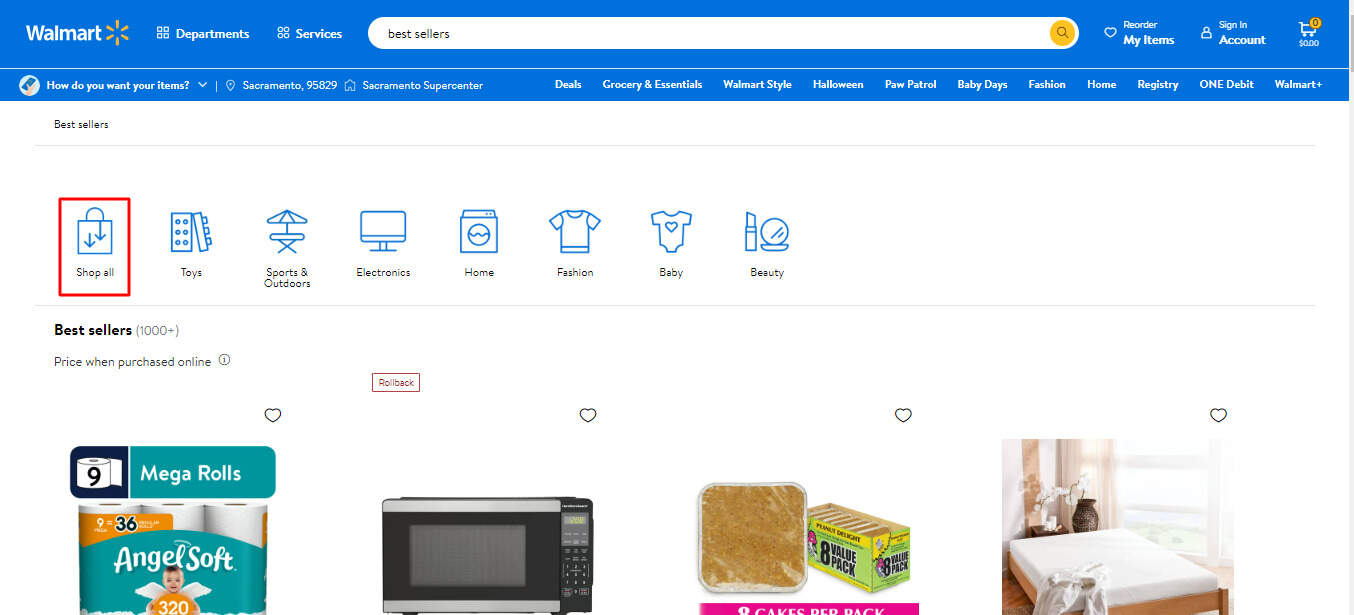This image features the Walmart homepage, prominently showcasing the signature blue header adorned with the Walmart logo, accompanied by the iconic gold flower insignia. Centered within the header is a versatile search bar, inviting users to look up various items. To the right, user navigation options are visible, including a "My Items" section, a prompt to "Sign In to Your Account," and a shopping cart icon marked with an orange circle displaying the number of items in the cart.

Beneath the header, a series of interactive prompts and categories are displayed, helping users tailor their shopping experience. Users are asked, "How do you want your items?" and can explore various categories including Deals, Grocery Essentials, Walmart Style, Halloween, Paw Patrol, Baby, and additional options extending to the right.

Further down, the site features specific shopping sections such as Toys, Sports, Electronics, Home, Fashion, Baby, and Beauty, each represented by vibrant pictures. Highlighted product images include a pack of Angel Soft Mega Roll toilet paper, a microwave, and a cut-off image that likely represents an eight-pack of coffee cakes. Also featured is a neatly arranged image of a bedroom, emphasizing Walmart's diverse product offerings.